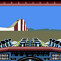This is a very small thumbnail image, likely from a computer game, measuring about one inch by one inch or smaller. At the top, there is a horizontal strip that transitions from dark brown to light brown, along with a noticeable red section. Below this, there is a large area of bright blue that represents the sky. Towards the left, there is a reddish-yellow structure, potentially a barn or a church, with a bit of white behind it. This is situated on the horizon where the green field meets the blue sky. Surrounding the scene are gray railings, with a prominent red railing running horizontally from left to right. At the front and back ends of the image, additional gray elements are visible. The bottom part of the image features two blue semicircles and strips of black and gray, possibly part of a high-tech vehicle's dashboard.